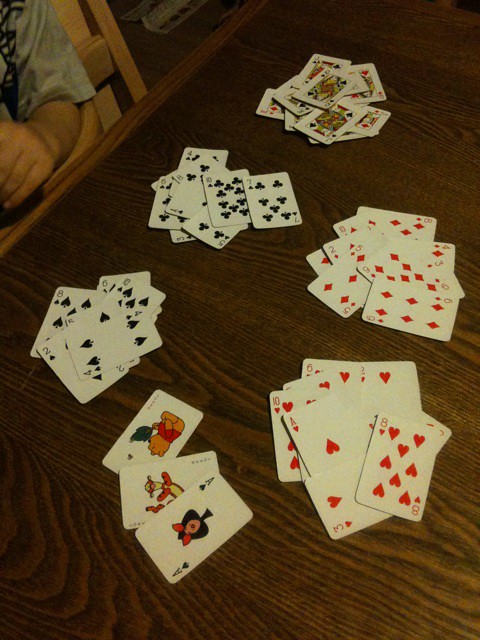A close-up of a beautifully crafted brown wooden table with intricate green and darker brown wood patterns dominates the image. In the upper left corner, a person's hand is visible, resting near the edge of the table. This person is sitting on a chair positioned beside the table and is focused on a set of playing cards arranged in front of them. 

The table holds five distinct stacks of cards. The first stack, situated in the upper left, comprises royals and special cards, including kings, queens, and jokers. Adjacent to it, the second stack displays a collection of clubs. The third stack features all the black aces. Moving further right, the fourth pile consists exclusively of red diamonds. Finally, the fifth stack showcases red hearts, with an additional ace peeking out from the bottom. The careful sorting of these cards suggests a game in progress or meticulous organization. The scene encapsulates a moment of quiet engagement and concentration.